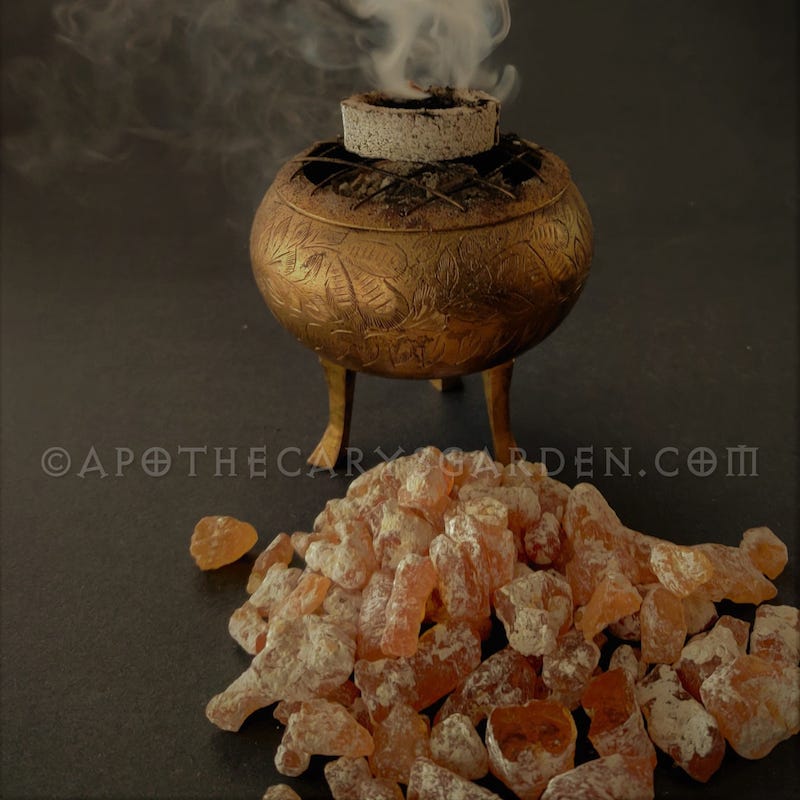This photograph, sourced from apothecariesgarden.com, features an ornate brass incense burner with three legs and intricate leaf carvings, prominently displayed against a dark gray background. The spherical incense burner has a piece of lit cake-style incense on top, with delicate tendrils of smoke curling into the backdrop. Across the middle of the image, in a distinctive runic-style font, is a watermark reading "© apothecariesgarden.com," where the O's are stylized as circles with crosses inside, contributing to a Nordic or runic aesthetic. In the foreground, there are chunks of pink, salt-like mineral rocks, covered in a powdery white coating, adding texture and contrast to the scene. The image is softly lit, creating a warm and inviting atmosphere.